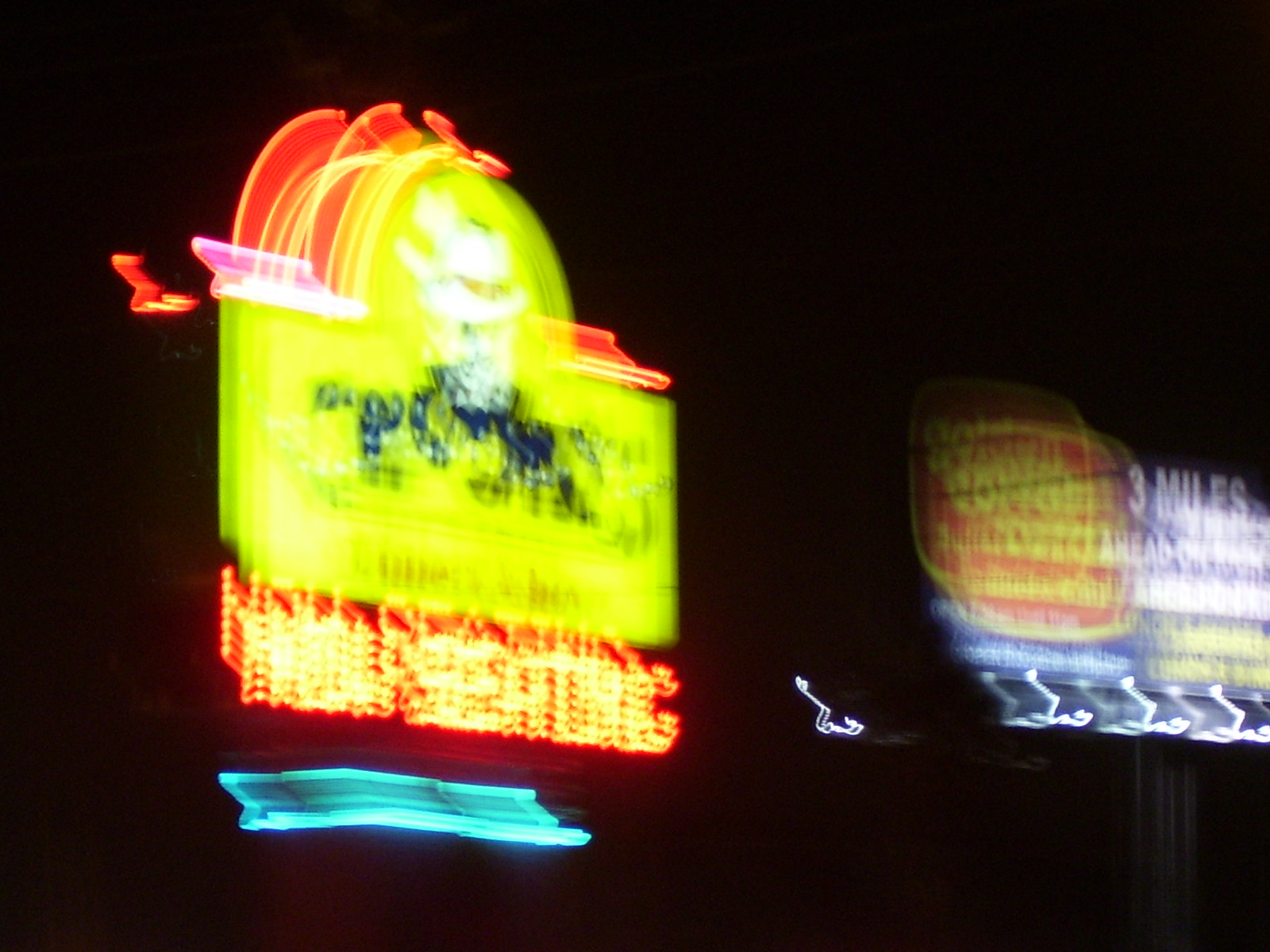This nighttime photograph features two prominent, yet blurry and distorted, street signs against a pitch-black background. The sign on the left appears to be a restaurant's neon sign, predominantly yellow with orange highlights, forming a shape that arcs upwards into a half-circle and back down. A white figure, possibly a character, is situated within this arc. Below this, a red section displays the words "Now Seating" in bright white lights, and beneath that lies a small strip of blue light, likely composed of several glowing tubes.

To the right of this, there is a large billboard, possibly for a Golden Corral, though its details are indistinct. This billboard features a disjointed red background with yellow lettering on one side and a darker blue section with white text indicating "Three Miles Ahead." The individual light fixtures on the billboard are faintly visible amid the generalized blur of the image.